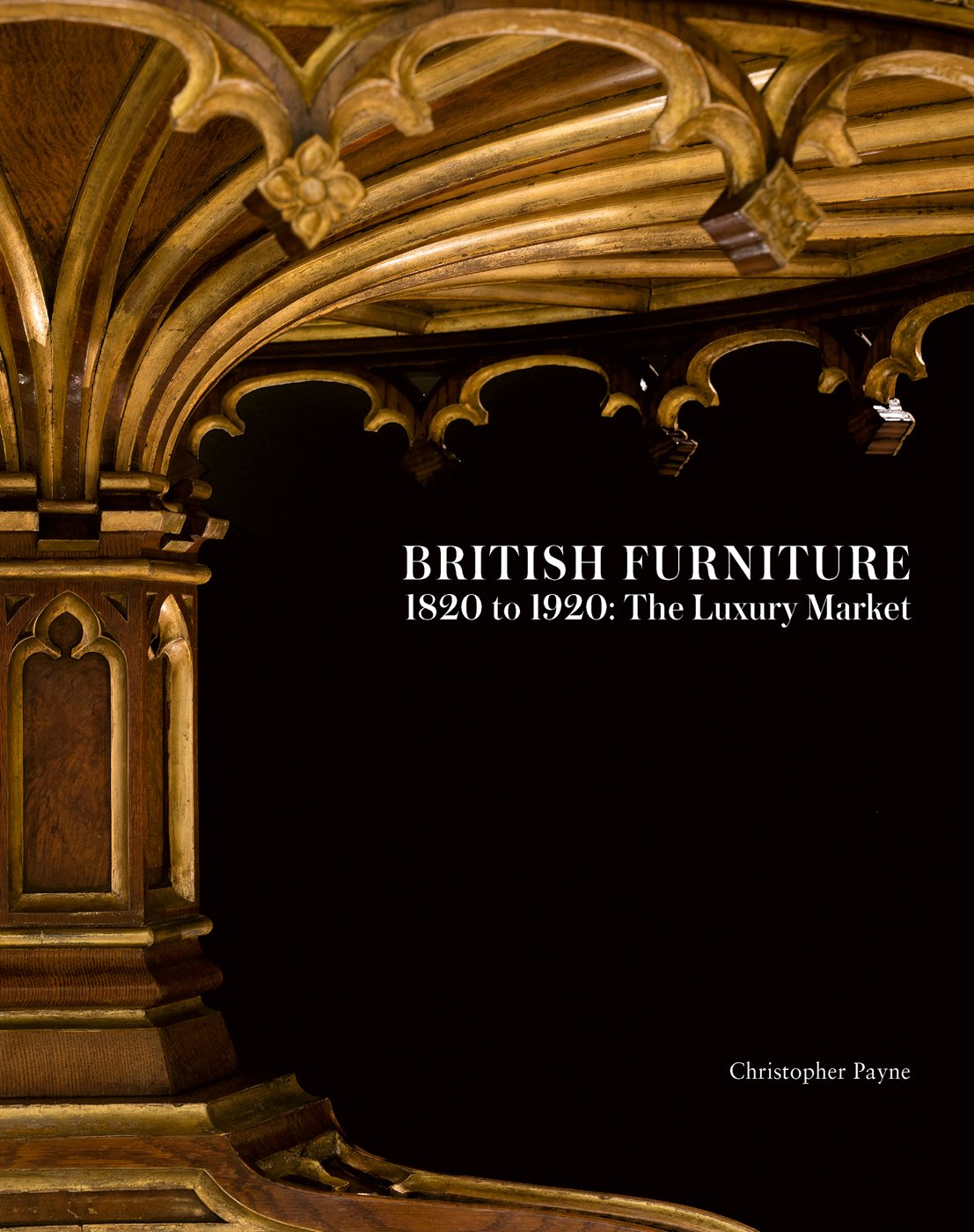This vertical image appears to be the front cover of a book titled "British Furniture 1820-1920: The Luxury Market" by Christopher Payne. The cover features a stark black background with the title and author's name displayed in a serif white font. Dominating a significant portion of the cover is a realistically taken photograph of an ornate wooden table, likely made of light brown wood. The photograph presents a detailed view from beneath the table, highlighting the elaborately carved underside. Visible elements include the bottom surface of the table, the central supporting column on the left, and one of the legs along the bottom. The intricate carvings on the table's edge feature dangling curlicues that end in floral designs, showcasing the luxury and craftsmanship of British furniture from the period.